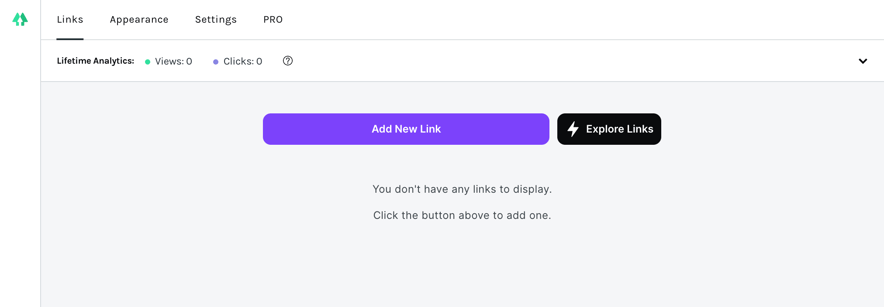The screenshot features a user interface with several distinctive elements. On the very left-hand side, there is an icon resembling two pine trees. Moving across the header bar, there are several tabs: "Links," which is currently selected, followed by "Appearance," "Settings," and "Pro PRO." Underneath the tabs, a white rectangle displays the text "Lifetime Analysis." Next to this, a small green circle indicates "Views 0," and beside it, a small purple circle shows "Clicks 0." There is also a question mark icon within a circle for additional information.

On the far right side of the header bar, there is a down-arrow button. Below the header, a large gray rectangle spans the width of the interface. Within this section, a prominent purple button labeled "Add New Link" is situated. To its right, a black button featuring a lightning bolt icon is labeled "Explore Links." Beneath these buttons, a message indicates, "You don't have any links to display," and a further instruction reads, "Click the button above to add one."